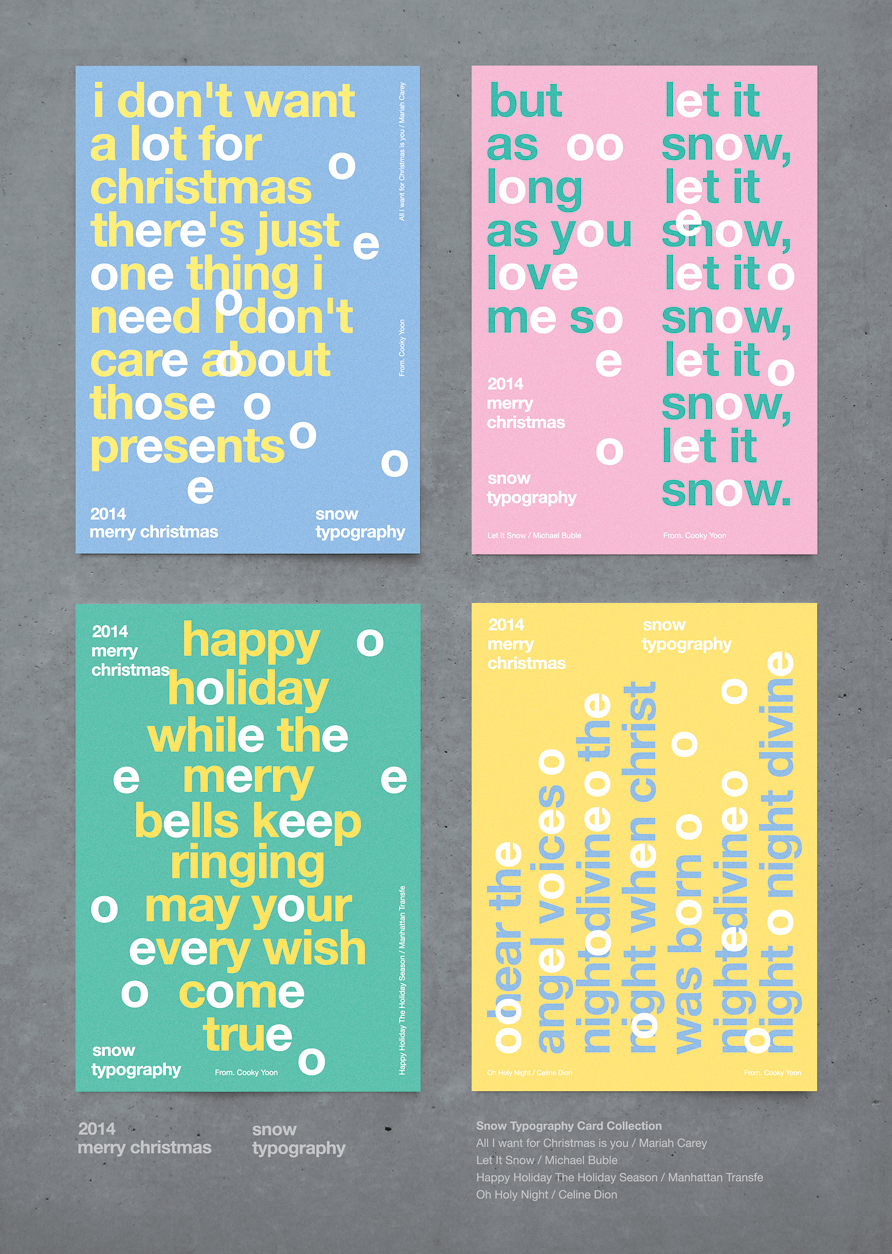This image features a set of four festive posters, all uniformly sized and set against a light gray background. Starting from the top left, the first poster is in blue with yellow and white text. It reads, "I don't want a lot for Christmas, there's just one thing I need, I don't care about those presents." Additionally, the words "2014 Merry Christmas," and "Snow Typography," are noted at the bottom right.

Moving to the upper right, there is a pink and green poster with white and green lettering that states, "But as long as you love me, let it snow, let it snow, let it snow." The corner includes the inscriptions, "2014 Merry Christmas," and a mention of "Snow Typography."

On the bottom left, the green poster with yellow and white text reads, "Happy holiday, while the merry bells keep ringing, may your every wish come true." This poster has "Snow Typography," at the bottom left and, "2014 Merry Christmas," written in the top left corner.

Lastly, the bottom right features a poster with text oriented sideways. It is primarily yellow with blue and white lettering that reads, "Hear the angel voices, night divine, when Christ was born, night divine, night divine." It also includes the text "2014 Merry Christmas," and "Snow Typography" in the top left corner. Each poster is part of the "Snow Typography" series and includes song credits for holiday classics, including "All I Want For Christmas Is You" by Mariah Carey, "Let It Snow" by Michael Buble, "Happy Holiday/The Holiday Season" by Manhattan Transfer, and "O Holy Night" by Celine Dion.